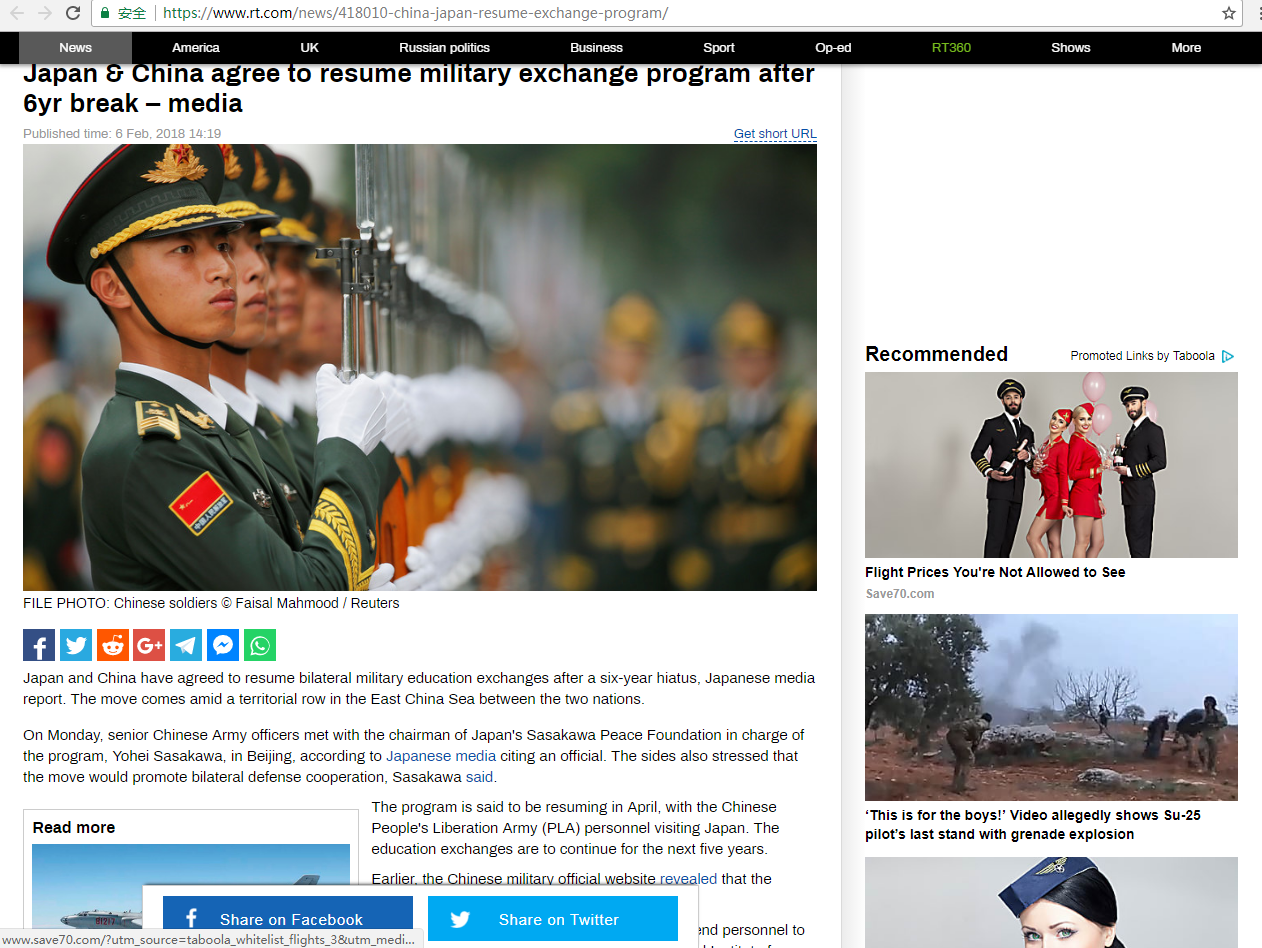**Detailed Caption:**

Japan and China have agreed to resume their bilateral military education exchanges, ending a six-year hiatus, according to Japanese media reports. This announcement comes against the backdrop of ongoing territorial disputes in the East China Sea between the two nations. The agreement was finalized during a meeting on Monday between senior Chinese army officers and the chairman of Japan's Sasakawa Peace Foundation in Beijing. The program, slated to restart in April, will involve personnel from the Chinese People's Liberation Army visiting Japan, and is planned to continue for the next five years. The goal of these exchanges is to enhance bilateral defense cooperation, according to statements from Sasakawa.

The accompanying file photo, captured by Fisal Mahmoud for Reuters, depicts Chinese soldiers equipped with rifles, affixed with bayonets, and clad in full military uniform complete with chin straps on their hats. 

Additionally, there are other images included in the news piece:
- The first image shows two captains, one holding balloons and the other a bottle of champagne, flanked by two stewardesses dressed in midi skirts and caps, both blonde. The caption for this photo reads, "Flights you're not allowed to see."
- The second image appears to be from a battlefield, possibly in Vietnam, filled with smoke and soldiers in combat attire. One soldier is seen assisting another. The caption for this photo reads, "This is for the boys: video allegedly shows SU-25 pilot's last stand with grenade explosion."